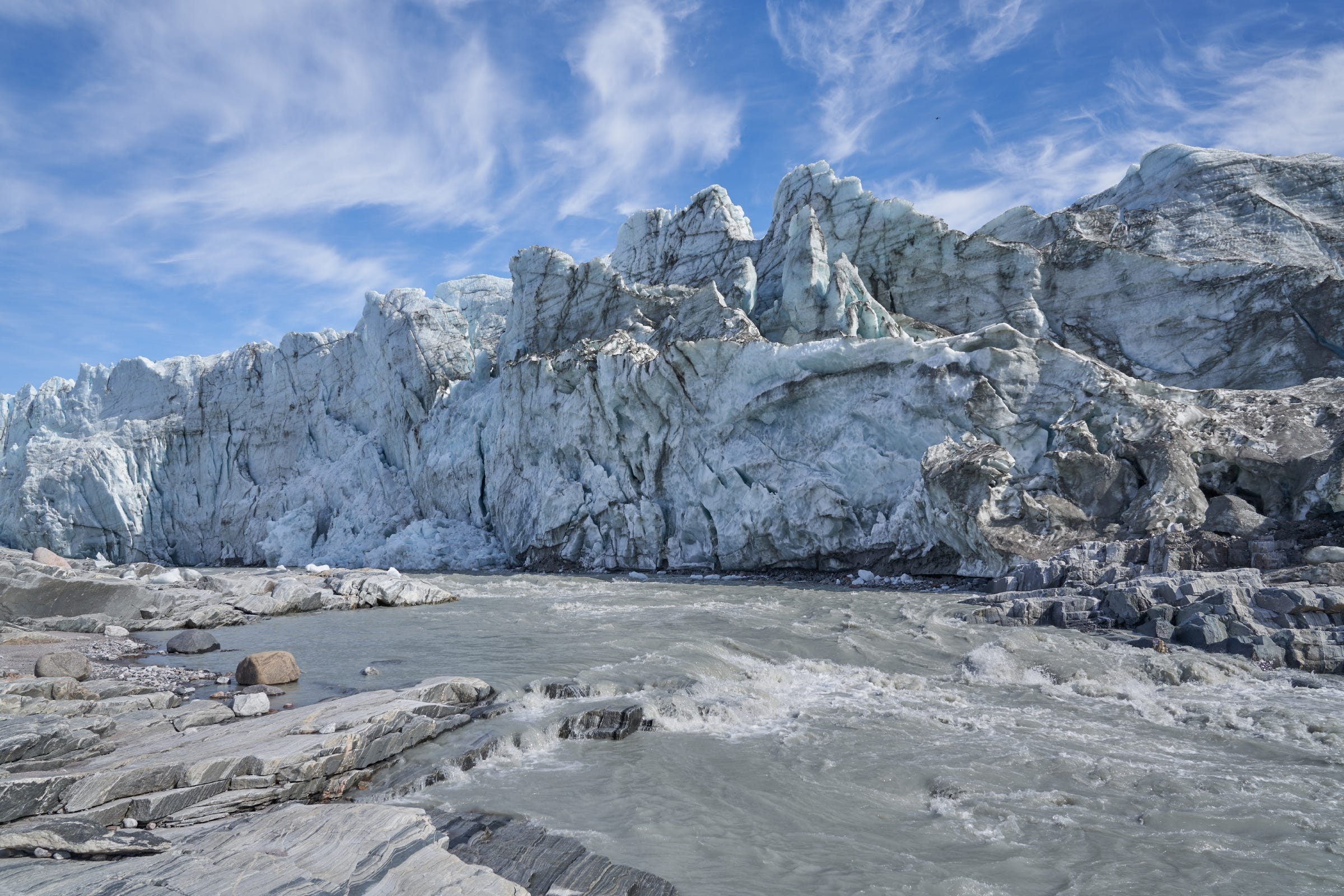This is a horizontal photograph taken outdoors during the day, featuring a dramatic, yet tranquil landscape. The scene captures a mountain range or perhaps a series of glaciers in the background, stretching horizontally from the left to the right edge of the image. These geological formations are a mix of light gray and white, suggesting they are partially snow-covered or composed of ice. The towering mountains or glaciers are jagged and rise steeply, creating a striking contrast with the clear, bright blue sky above. Wispy, transparent white clouds scatter across the sky, adding depth to the serene atmosphere. In the foreground, there is a rocky area consisting of flat, granite-like rocks, varying in shades of dark and light gray. These rocks appear snow-dusted and are situated beside a narrow, flowing river. The river, shallow and cold, rushes gently over the rocks, adding a dynamic element to the otherwise still scene. The photograph is bathed in natural light, though there's a noticeable shadow cast over parts of the glacier in the background, likely caused by the sun's angle.